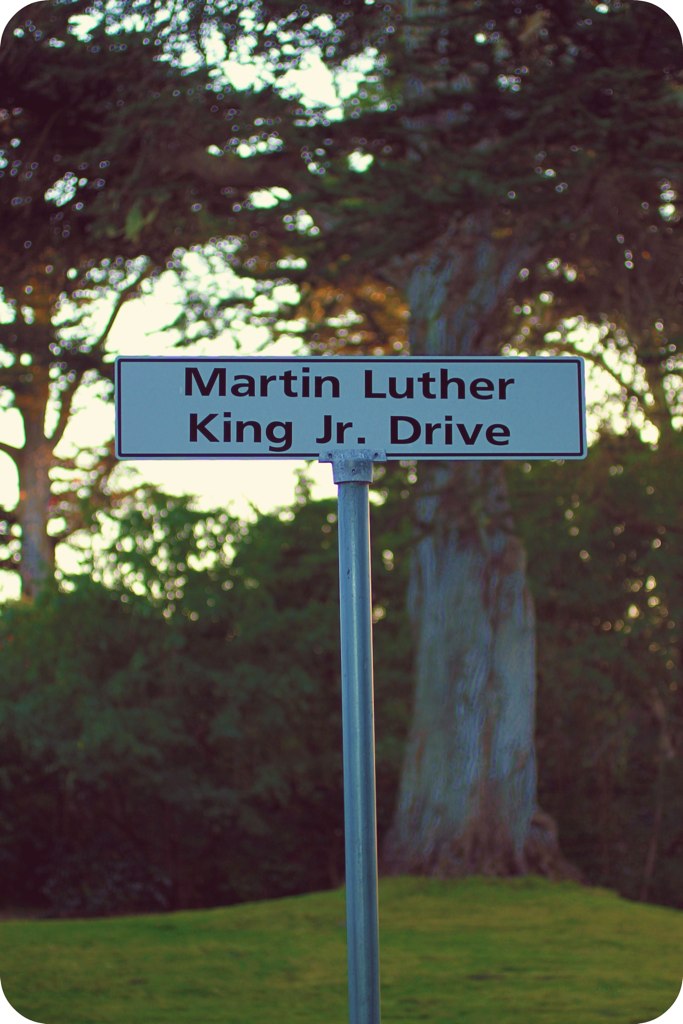A lifelike photograph capturing a street sign that reads "Martin Luther King Jr. Drive," affixed to a sturdy metal pole anchored into the ground. Behind the sign stand towering trees, their abundant foliage suggesting a scene set in either spring or autumn. Nestled below the trees are sizeable bushes or shorter trees, all thriving on a verdant carpet of grass interspersed with lightened patches. The natural sunlight, indicative of daytime, illuminates the scene, enhancing the vivid greenery and the tranquil yet vibrant essence of the setting.